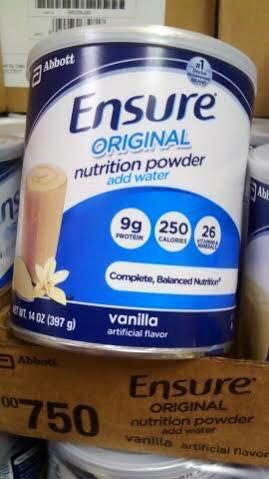The image is a close-up, first-person perspective photograph of an Abbott-branded can of Ensure Original Nutrition Powder, likely taken in a grocery store. The can's label is detailed with a dark blue top section, a white middle, and a light blue lower half in a semi-circular shape. The top left of the label features the Abbott logo, while the top right has a circle indicating it is the number one recommended brand, accompanied by small blue text. Prominently in the center, the label reads "Ensure Original Nutrition Powder" with "Add Water" following below. On the left side of the label, there is an image of a vanilla shake with a vanilla flower in front of it. Key nutritional information is displayed in three white circles on the light blue part of the label, highlighting "9g Protein," "250 Calories," and "26 Vitamins and Minerals." A white banner beneath these circles states "Complete Balanced Nutrition." At the very bottom of the can, it mentions "Vanilla Artificial Flavor" along with the net weight of "14 ounces" or "397 grams." The can, featuring a clear plastic lid, is situated in a cardboard case along with other identical cans. The case has the Abbott logo and "Ensure Original Nutrition Powder, Add Water, Vanilla" printed on it, reinforcing the context of a grocery store display.